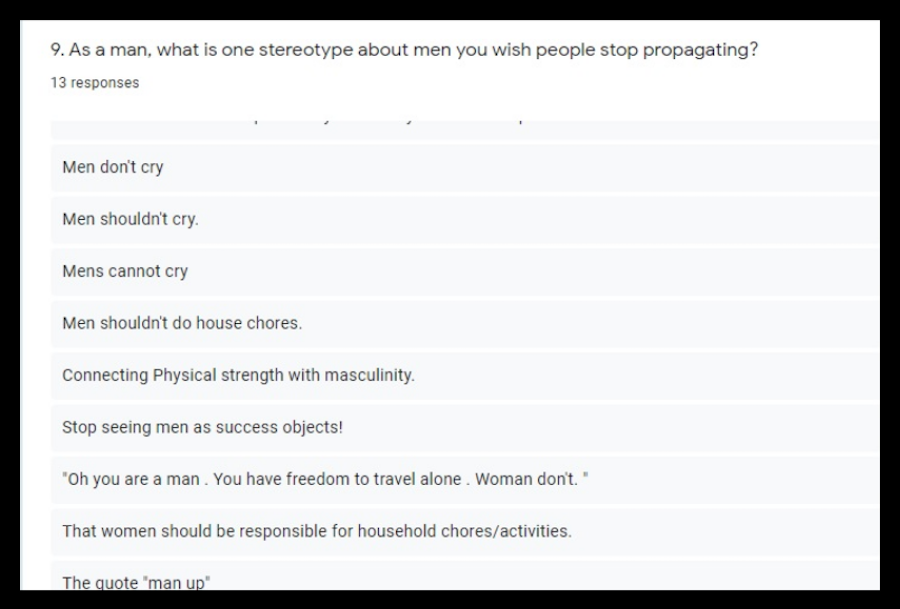A square image on a white background features several vertical rows of individual, long, thin, horizontal light gray boxes, each containing a response. The boxes have thick black borders and dark gray text inside. At the top, a black text reads, "9. As a man, what is one stereotype about men you wish people would stop propagating?" followed by "13 responses." Each response is contained within its own light gray box. The responses listed are as follows:
1. "Men don't cry."
2. "Men shouldn't cry."
3. "Men cannot cry."
4. "Men shouldn't do house chores."
5. "Connecting physical strength with masculinity."
6. "Stop seeing men as success objects!"
7. (In quotes) "Oh, you are a man. You have freedom to travel alone. Women don't."
8. "That women should be responsible for household chores and activities."
9. "The quote 'man up.'"